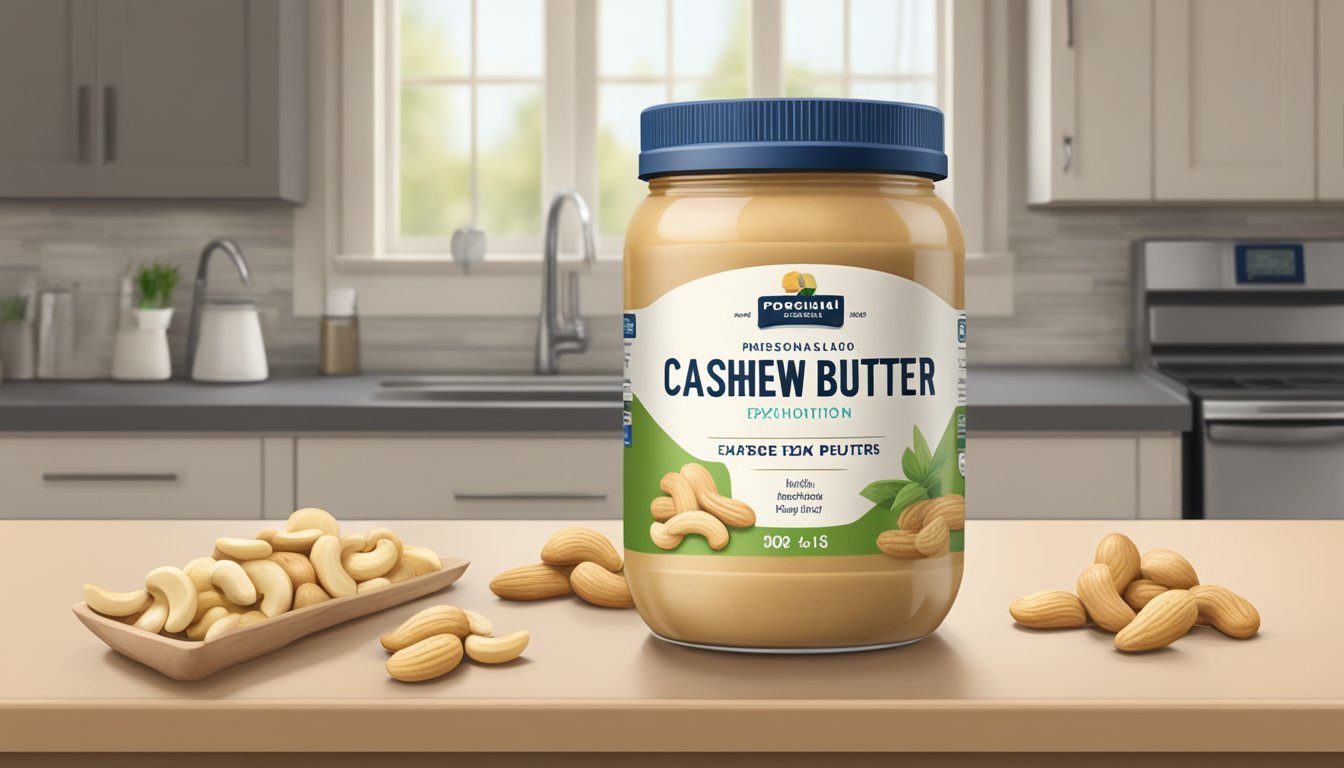The image captures a pristine, AI-generated kitchen scene primarily centered on a jar of cashew butter, positioned on a beige-colored island countertop. The kitchen radiates a modern aesthetic with its smooth gray counters and cream-colored cabinets, accessorized with stainless steel fixtures and decor. Behind the central jar, which is adorned in a green, white, and black label with a blue lid, sits a triple-pane window above a sink, whose faucet is slightly to the left of the jar. To the right of the sink, a stainless steel stove is accentuated by overhead cupboards, while to the left, a white kettle and ceramic pieces complement the scene. The countertop also features scattered cashews, including several in a tan oblong dish, arranged meticulously to highlight the purity and natural quality of the cashew butter. A tan-colored shelf in the forefront adds a warm touch to the otherwise sleek, contemporary kitchen, making the jar of cashew butter the clear focal point of this ad-like photograph.